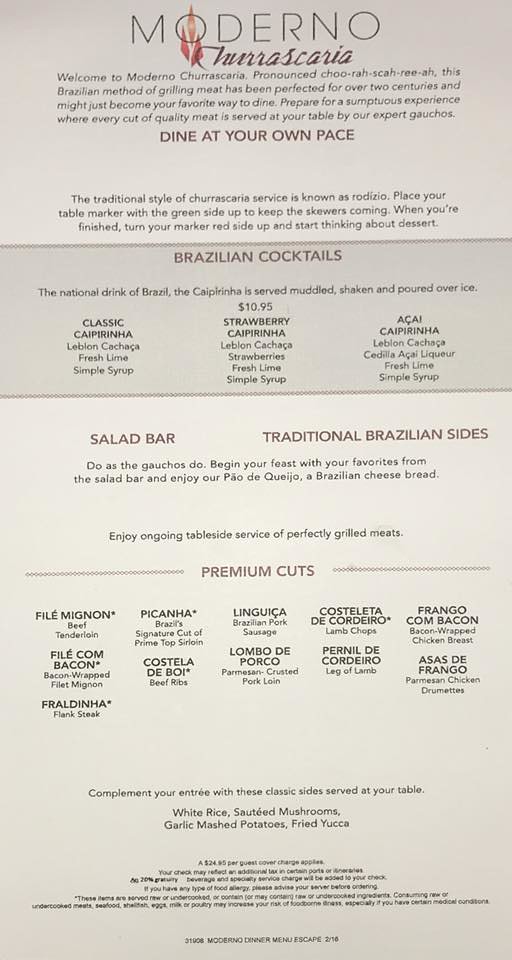Indoor color photograph of a menu for a Brazilian restaurant. The menu is printed on a long rectangular sheet of white paper. Starting at the top in capital, thin letters is the restaurant's name, "Moderno." Beneath it is a script font which reads "Churrascaria." A four-line paragraph follows, describing the restaurant's concept and ambiance. Immediately below, in larger bold letters, it states, "Dine at your own pace."

About a third of the way down the menu, there's a shaded rectangle featuring the heading "Brazilian Cocktails," which showcases three columns of various cocktails, each offering three to four different flavor options.

Returning to the white background, we see the left subheading labeled "Salad Bar" while the right side features "Traditional Brazilian Sides."

Near the bottom, a horizontal line separates the sections, with the heading "Premium Cuts" in the center. This section lists 10 different cuts of meats including beef, chicken, and lamb chops. Finally, at the very bottom of the menu, there's a section of fine print, which is illegible in the photograph.